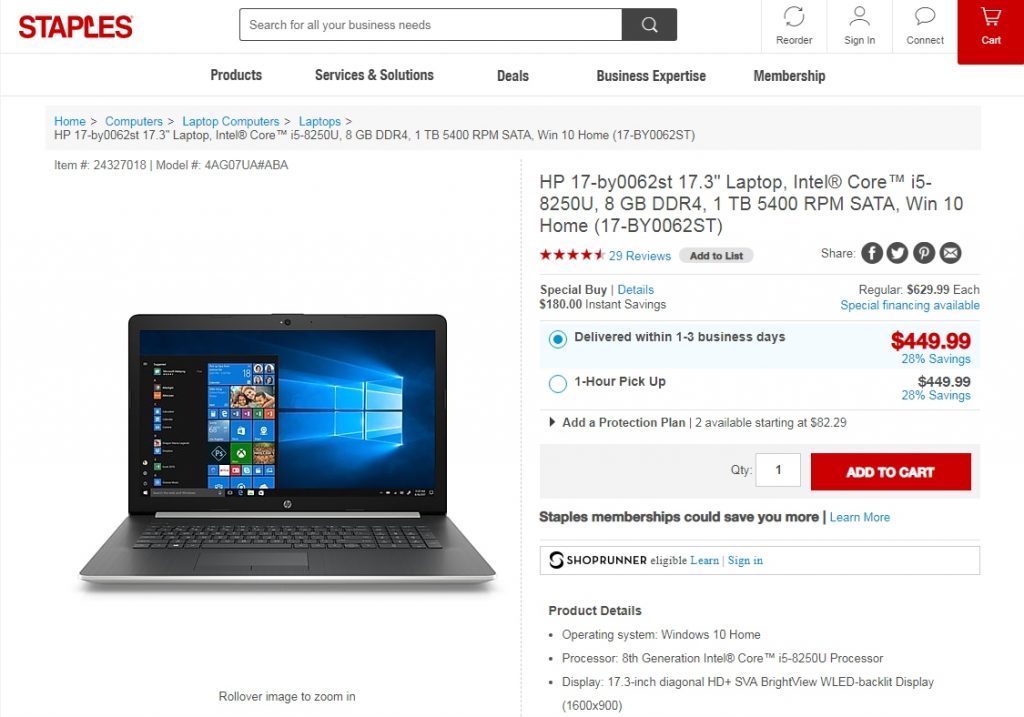The screenshot captures a product page from the Staples website. In the top left corner, the recognizable red Staples logo is prominently displayed. At the top of the screen, a convenient search bar reads, "Search for all your business needs," accompanied by a grey search button featuring a magnifying glass icon. Proceeding to the top right, there are several functional buttons labeled "Reorder," "Sign In" with a small person icon, and "Connect" with a chat icon. A red button labeled "Cart" includes an icon of a shopping cart. 

Below these, a navigation menu presents various options, including "Products," "Services and Solutions," "Deals," "Business Expertise," and "Membership."

The product showcased on this page is a laptop, evident in the left section of the screenshot by a detailed product photo. The laptop appears to be a Windows device, as indicated by its screensaver displaying the iconic Windows logo with blue light emanating from the "window." 

On the right side, the product details specify the laptop's model and specifications: This HP 17-BY0062ST features a 17.3-inch screen, an Intel Core i5-8250U processor, 8GB DDR4 memory, and a 1TB 5400 RPM hard drive.